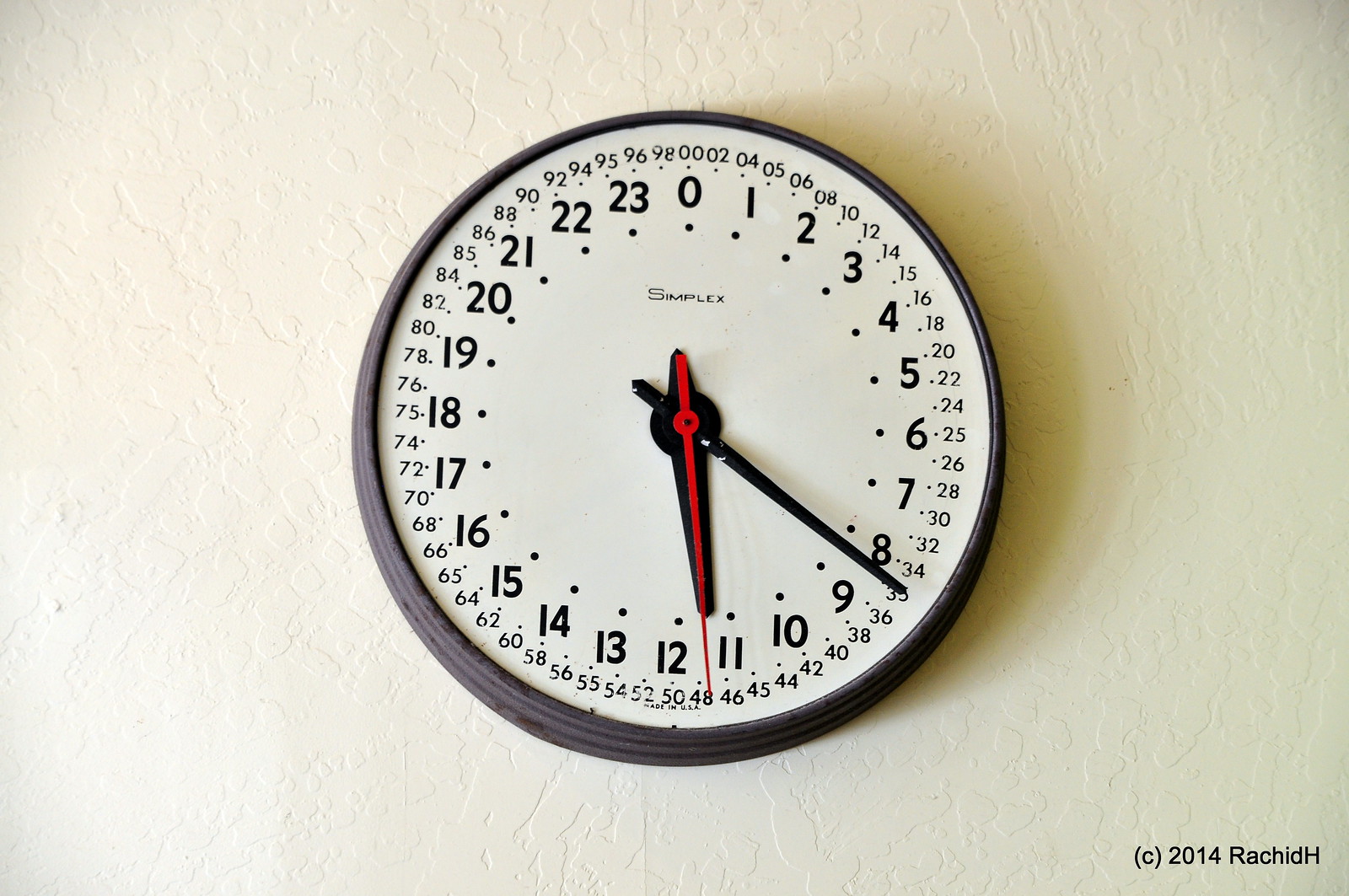This is a detailed color photograph of a unique 24-hour wall clock mounted on a white wall. The round clock has a white face and is encased in a black or possibly grayish frame, which may or may not have a glass cover. The clock features a black, thick, and short hour hand, a long, thin black minute hand, and an even longer, skinny red second hand.

The clock displays hours in a 24-hour format, starting from zero at the top and going clockwise to 23. On the inside edge of these numbers are small dots indicating precise positions. Additionally, there are more increments around the clock for seconds, numbered from 0 to 100 in pairs, such as 2, 4, 6, and so forth, ending at 98, with double zeros at the top.

In the lower right-hand corner of the clock, there is a copyright mark reading "(C) 2014 RACHID H." The brand name "Simplex" is also noted. This clock operates on military time and provides a distinctive way of tracking time with its incremental and detailed design.